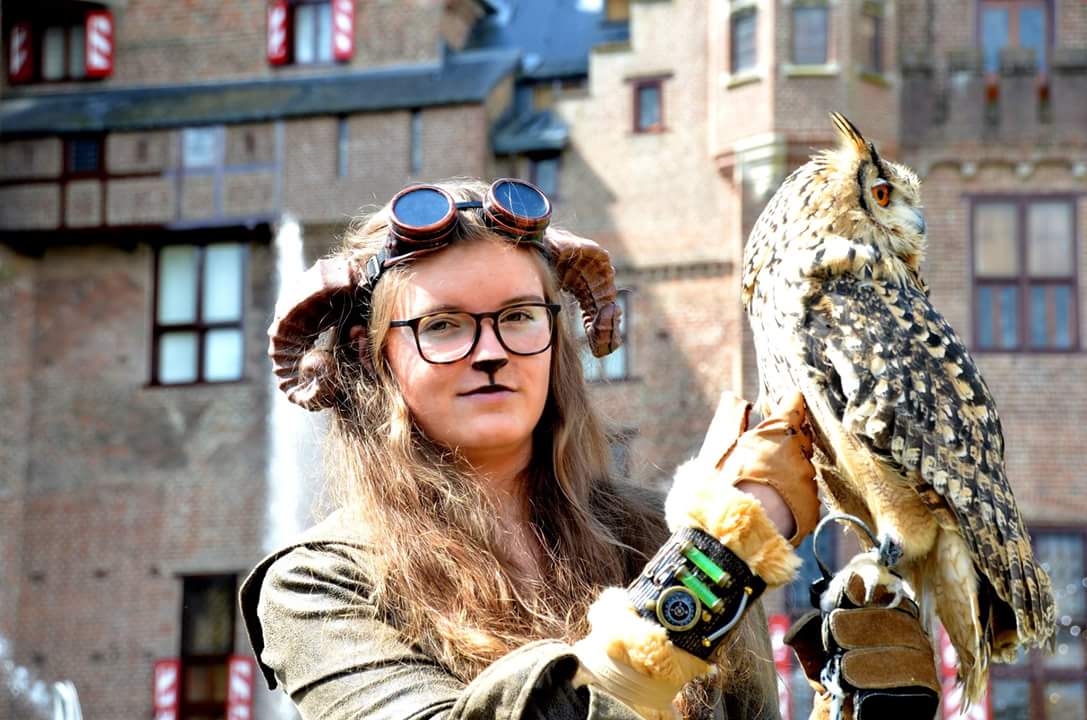In the vibrant outdoor scene, a multi-story building with tan and red bricks serves as the backdrop, bathed in sunlight. The building features an array of windows—some large and some small, with varying window panes. A distinctive rounded section on one side gives the impression of a separate room, accented by red elements that might be shutters or a sign.

The main focus is a young woman standing confidently in the foreground, clearly engaging in cosplay. She wears a pair of elaborate steampunk goggles atop her head, alongside faux horns akin to those of a doll sheep. Her long, flowing blonde hair cascades down past her arms, complemented by black-framed glasses. A drawn-on cat-like mark adorns the area below her nose, giving her a whimsical appearance. 

Dressed in a green sweater under a thick overcoat, she sports a unique wristband on her right wrist featuring green accents and fur detailing, in line with her steampunk theme. On her left hand, she wears a sturdy brown and black leather glove, on which an owl is perched. The owl, with its head turned to the right, has a striking mix of black and cream feathers, a light brown belly and head, and piercing orange eyes. The owl's black beak and sizable presence add to the visual intrigue.

Her right hand gently strokes the owl, creating a harmonious connection between the cosplayer and her avian companion as they both face the camera.